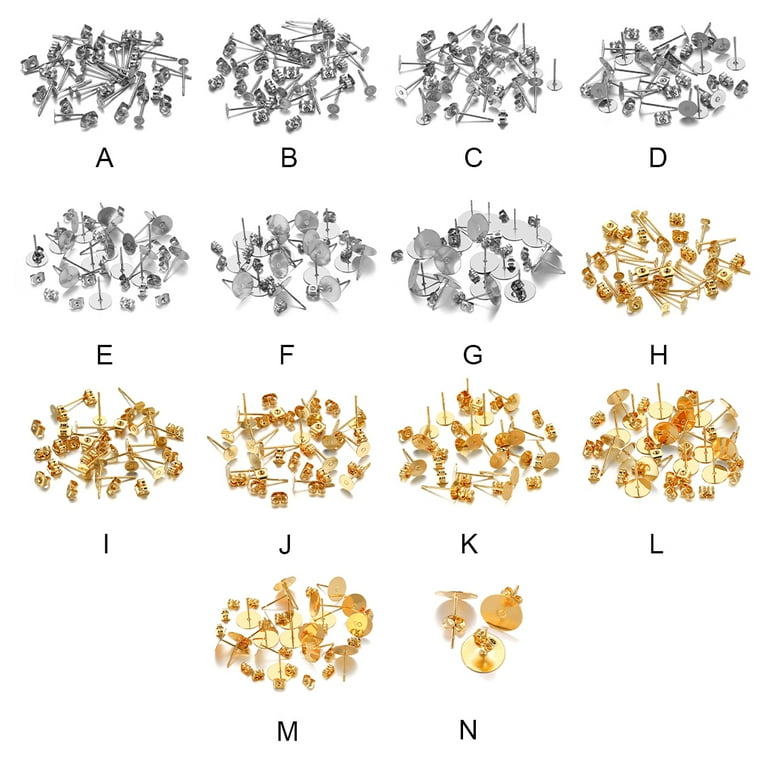The image displays a collection of various earring backings against a white background, meticulously organized and labeled from A to N in black text. The first seven groups, labeled A through G, feature silver backings, including standard backings and types with plastic inserts to prevent loss. The next seven groups, labeled H through N, consist of similar gold backings, with H through K showcasing typical yellow gold backings, and L through N featuring those with plastic inserts for added security. Each group displays a slightly different design, size, and function, providing a comprehensive catalog-like presentation of earring posts and backings.